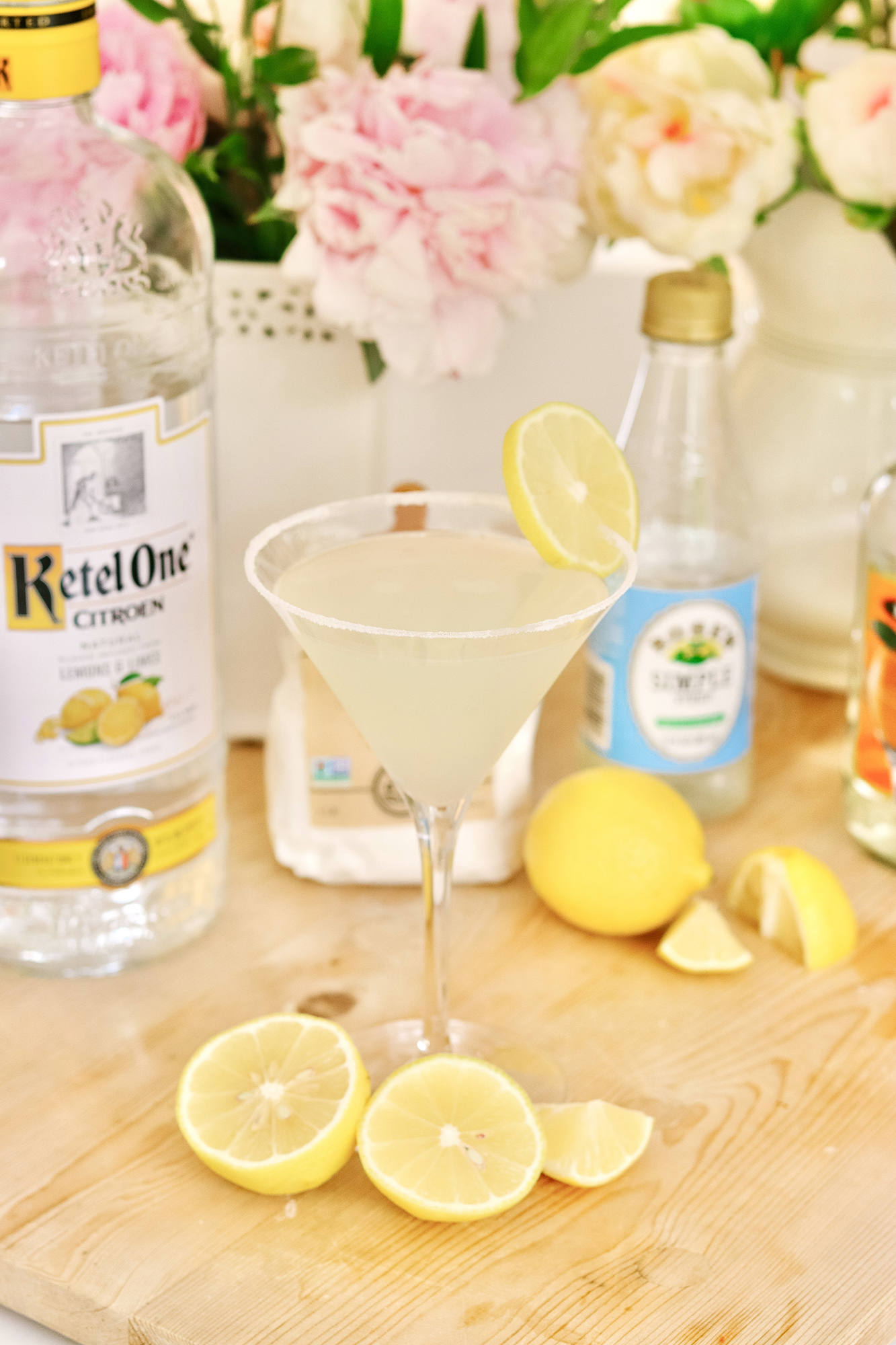The photograph captures a mixed alcoholic beverage, likely a spiked lemonade, elegantly served in a clear wine or cocktail glass with a sugared rim. The drink, a pale yellow liquid, is garnished with a slice of lemon. The glass is set on a wooden table, accompanied by fresh lemon slices and a whole lemon. The Kettle One Citron bottle, known for its lemon-flavored vodka, sits prominently on the left, indicating the presence of vodka in the lemonade. Surrounding the scene, powdered sugar and other mixers, including a bottle with an orange label and another with a blue label, can be observed. In the backdrop, vibrant florals in white vases add a decorative touch, featuring light pink and yellow carnations.